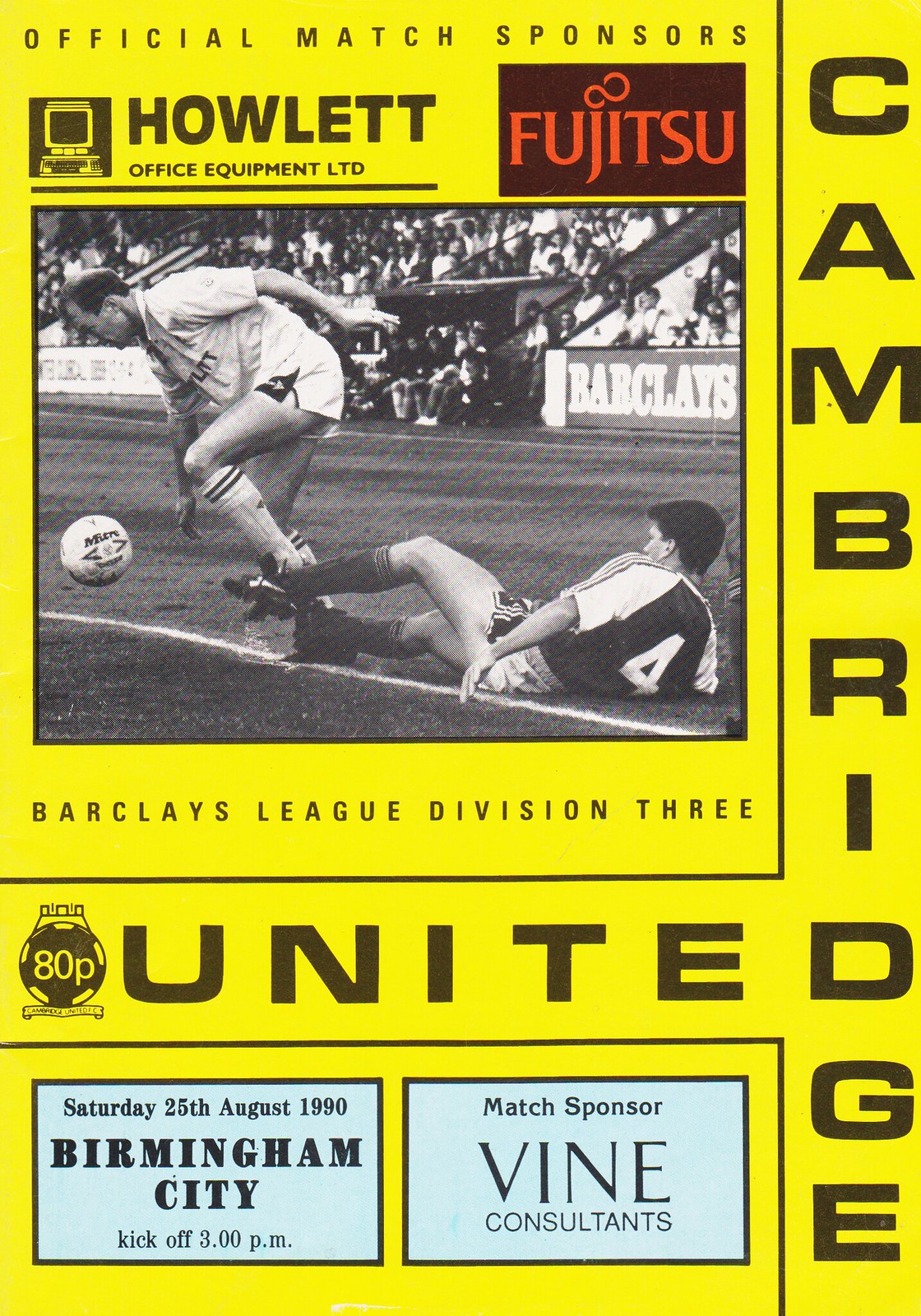The image displays a vibrant yellow program cover for a Barclay League Division 3 soccer match. At the very top, "Official Match Sponsors" is printed. Below, on the left side, there is an illustration of an old-fashioned computer next to the name "Howlett Office Equipment Limited." Positioned to the right, the name "Fujitsu" is prominently featured in red text. Central to the image, a black and white photograph captures an intense moment during a soccer match, with one player attempting to tackle another while the ball is loose on the ground, against the backdrop of a large audience. Beneath this action shot, the text reads "Barclays League, Division 3." The words "Cambridge" and "United" are printed vertically and horizontally, respectively, intersecting at their shared "D." At the bottom of the program, details are provided: "Saturday, 25th August 1990, Birmingham City, Kickoff at 3pm," with the match sponsored by Vine Consultants.